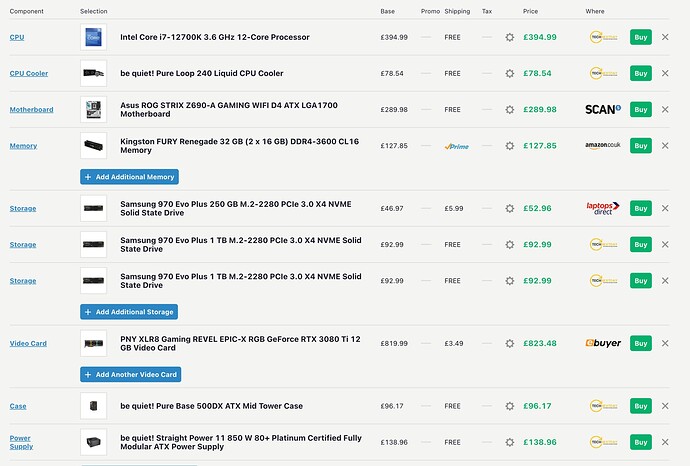The webpage features a comprehensive list of electronics products available for purchase, displayed on a light gray background. At the top of the screen, there are various category headings: "Component," "Selection," "Base," "Promo," "Shipping," "Tax," "Price," and "Wear."

On the left-hand side, under the "Component" column, a vertical list of options is presented in bright blue text. Adjacent to this, under the "Selection" column, is a detailed vertical list of product names, each accompanied by an image in black text.

In the "Base" column to the right, product pricing is indicated in pounds. The "Promo" column provides promotional information, while the "Shipping" column often displays "free" shipping options. Some entries feature the bright blue Amazon Prime logo, indicating Prime shipping. For other products, shipping costs range between four to six pounds.

Further to the right, the "Price" column showcases product pricing in bright green text. Lastly, in the "Wear" column, various pieces of information are listed. Each entry in this column is followed by a green "Buy" button, with the text displayed in white, inviting customers to make a purchase.